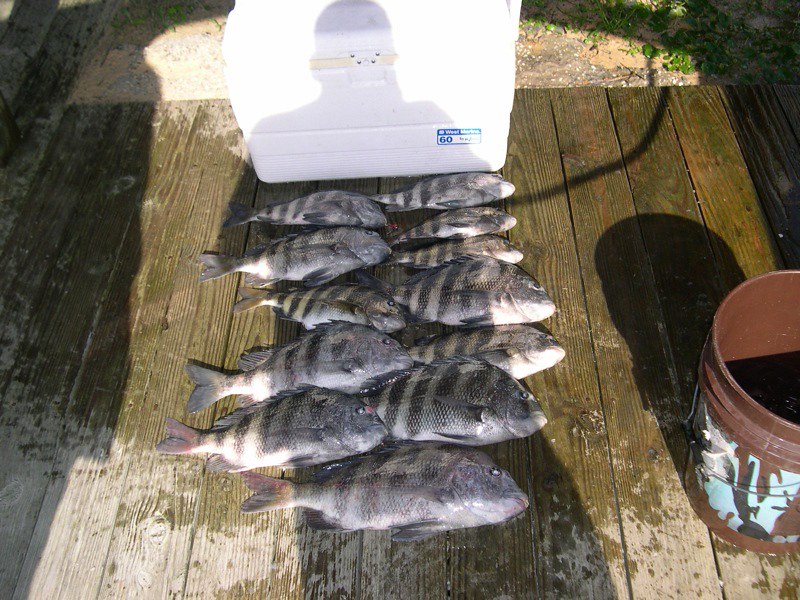This photograph captures an outdoor scene featuring freshly caught fish meticulously laid out on a wet wooden surface, possibly a pier or board. There are about 10 to 12 fish of varying sizes, arranged from the biggest to the smallest. On the right side of the wooden board, an empty brown bucket is visible. Behind the fish, there's a closed white cooler, likely used for storing the catch. The image is infused with a sense of human presence; the shadow of the person taking the photo is cast over the fish, adding a subtle layer of narrative. Beyond the wooden surface, the ground transitions into a dirt area interspersed with patches of grass and vegetation.